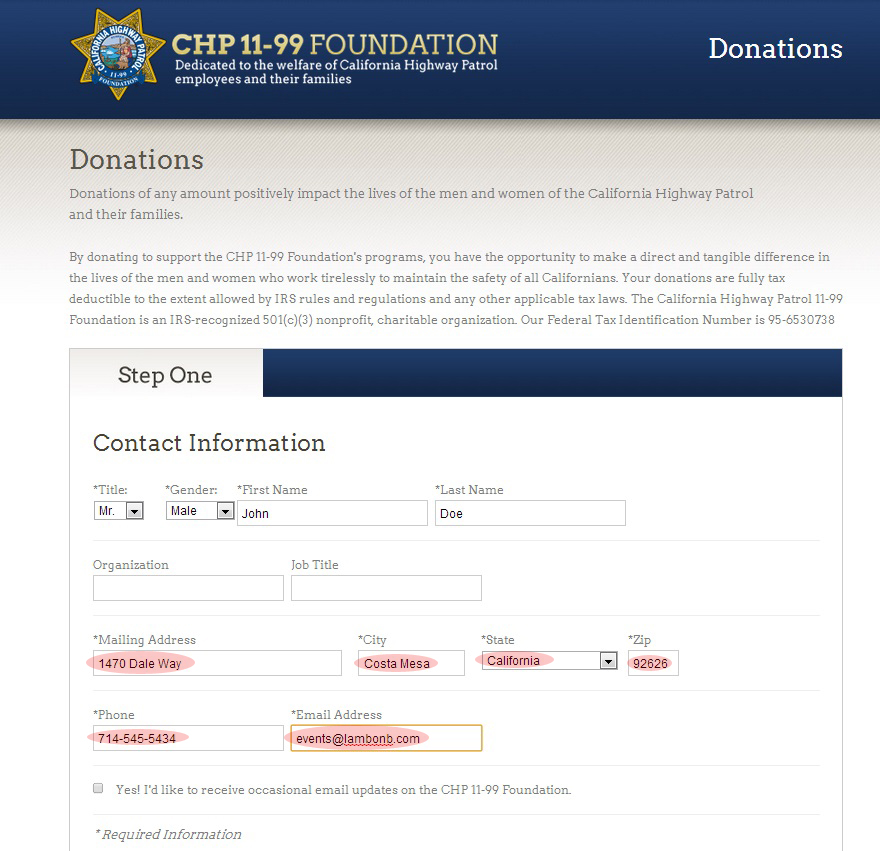The image is a contact information screen for the CHP 11-99 Foundation, displayed as a donation page from a website. At the top, there's a blue banner with the California Highway Patrol badge and the title "CHP 11-99 Foundation" which is dedicated to the welfare of California Highway Patrol employees and their families. The banner also features a brief description highlighting that donations of any amount positively impact the lives of CHP employees and their families by supporting the foundation's programs.

Below this banner, there's a white section titled "Donations" with instructions that request step one of the donation process—entering contact information. The screen includes various fields for personal details such as title, gender, first name, last name, organizational title, mailing address, city, state, zip code, phone number, and email. Partially filled information is evident; for instance, the title is marked as "Mr." indicating the gender is male, with the name "John Doe" entered. The mailing address is partially completed, showing a location in Costa Mesa, California. The contact information fields are emphasized with large pink ovals around them.

Additionally, there is a detailed message explaining that donations make a direct and tangible difference in the lives of CHP employees who work tirelessly to maintain the safety of all Californians. It mentions that the donations are fully tax-deductible to the extent allowed by IRS rules and regulations, and the foundation is recognized as a 501(c)(3) nonprofit charitable organization with the federal tax identification number 95-6530738.